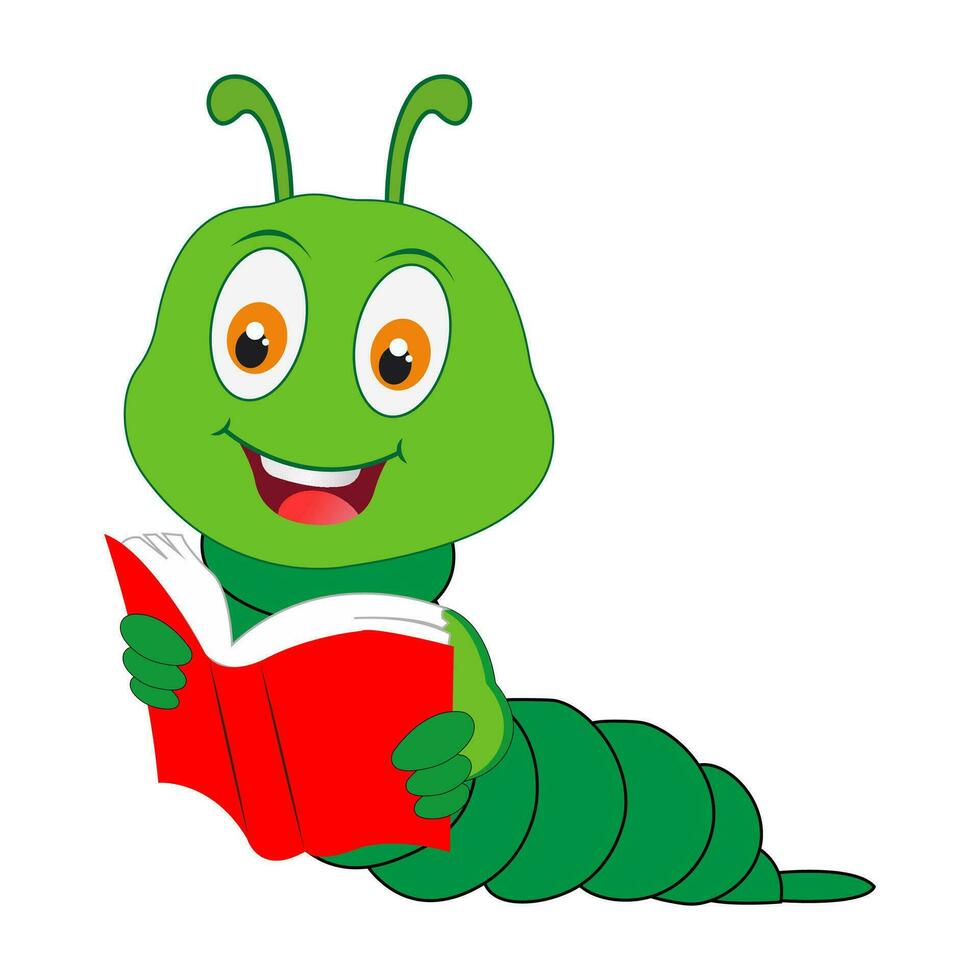The image features a cartoon caterpillar with a predominantly dark green body and a slightly lighter green head, which is disproportionately large compared to its body. The body trails off to the left, making it look like the caterpillar is in a playful, upward-leaning pose reminiscent of Superman. The character has two small green antennae extending upward and curving outward. 

The caterpillar's wide, expressive eyes consist of multiple colors: a white outer part, an orange middle section, black pupils, and small white highlights, giving the eyes a shiny, bright appearance. The caterpillar's mouth is open in a joyful smile, displaying a horizontal white bar that represents the top row of teeth, and a red tongue can be seen inside.

In his three-fingered hands, which are darker green than the arms, the caterpillar is holding an open red book filled with white pages. The scene is set against a plain white background, emphasizing the caterpillar's joyful interaction with the book.